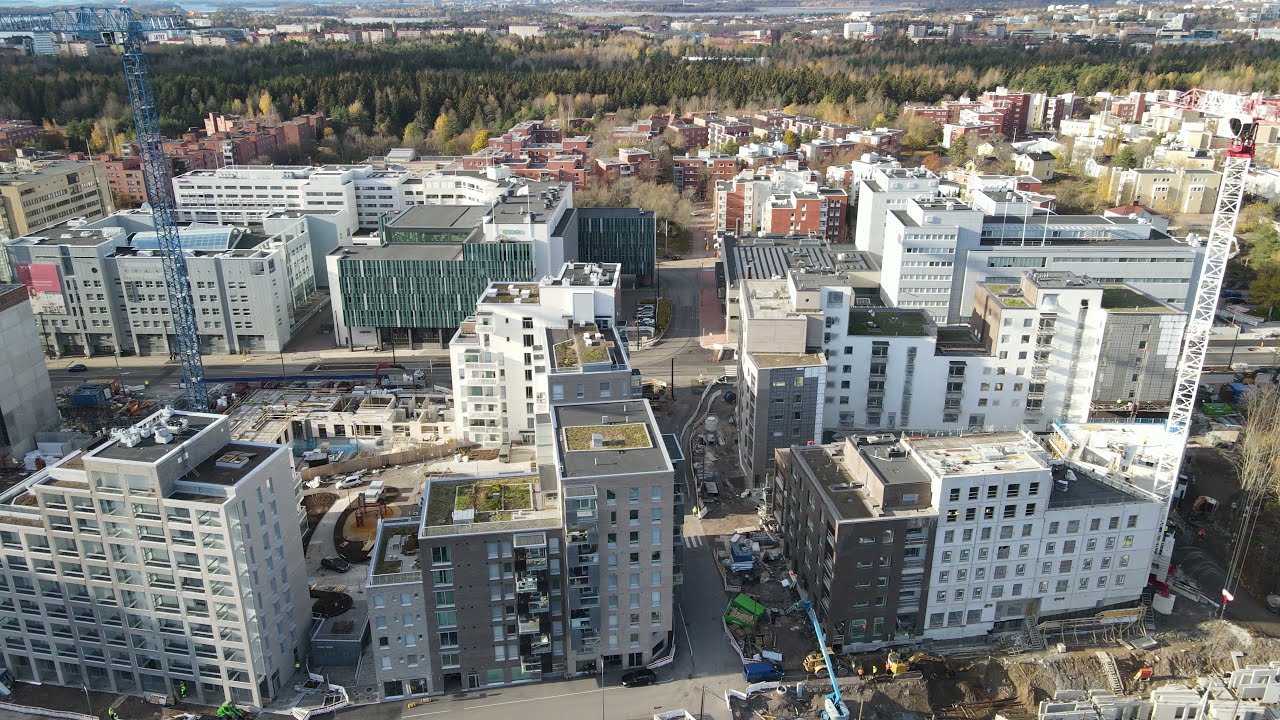This image provides a detailed drone shot of an industrial city abundant with diverse buildings and active construction sites. The foreground, dominated by buildings varying from 10 to 20 stories high, showcases a significant amount of ongoing construction, particularly noticeable in the bottom right where new buildings are being erected and roads are being worked on. This bustling construction area features cranes, including a prominent blue crane on the left and an orange structure on the center right. 

The buildings, made of different materials and colors, range from white to dark gray and light reddish hues, with some having extensive glass window constructions. Moving towards the middle of the image, the density of the buildings continues, with many appearing to be apartment complexes rich in windows and varying in design.

At the top of the image, about 20% of the space is filled with a forested area, displaying a palette of autumn colors—dominantly green, but interspersed with brown, yellow, and beige. Beyond this lush green canopy, in the far background, another cityscape emerges, marked by a scatter of smaller buildings that blend with the horizon, indicative of a sprawling urban expanse. This layered composition of built and natural environments offers a vivid and dynamic glimpse into the heart of an industrial urban landscape in the midst of growth and development.